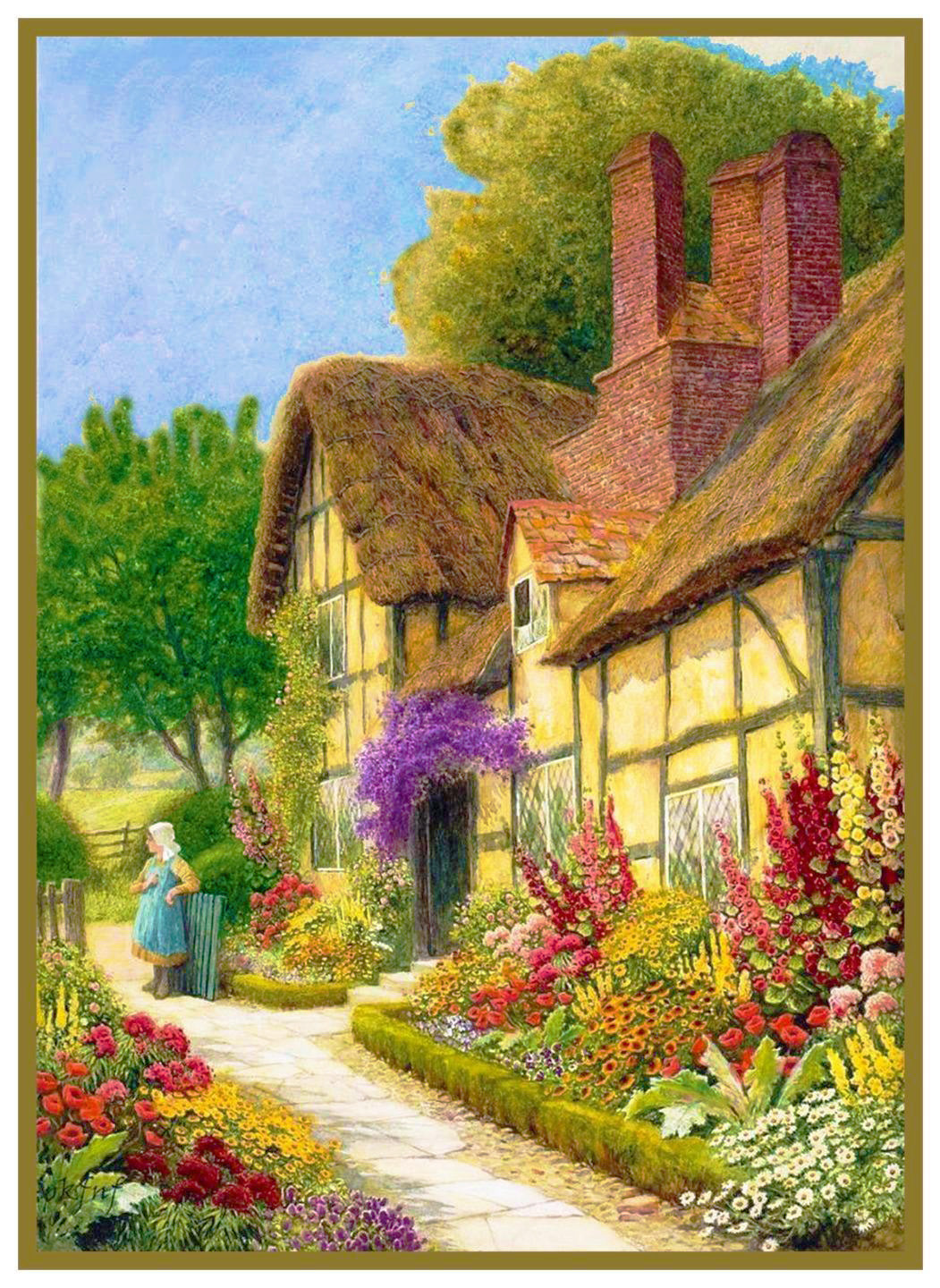The image is a detailed painting of an outdoor scene featuring a quaint, old-fashioned cottage with a distinct thatched roof and a large, red-bricked chimney stack. The cottage’s walls appear to be either orange or yellow, suggesting the use of warm earthy tones like stone or mortar. In the foreground, a variety of flowers—red, yellow, pink, purple, and white—create a profusion of color, with tall and short blooms arranged in wild beds. A small, stone pathway meanders through these vibrant flower gardens, leading up to the house. 

On the front of the house, there are three double windows on the bottom floor and a double window on the top floor, next to the chimney stack. Above the front door, which is reached by three steps, grow large pink and purple flowers, adding to the picturesque charm of the setting. 

Toward the bottom left corner, an array of deep red, purple, and orange flowers add further depth to the garden scene. A small wooden gate, painted blue, stands in front of the walkway, leading you further into the painting.

A young woman, or perhaps a girl, dressed in a blue apron over a yellow dress, is leaning against this blue gate in a relaxed pose. She wears a white bonnet and her profile is turned right to left, looking away from the house. Behind her, additional pathways stretch towards the cottage, where trees and a clear blue sky with a single white cloud complete the serene, pastoral scene.

The composition is surrounded by a subtle brown-green border, framing the idyllic landscape and drawing the viewer's eye into this tranquil, country setting.